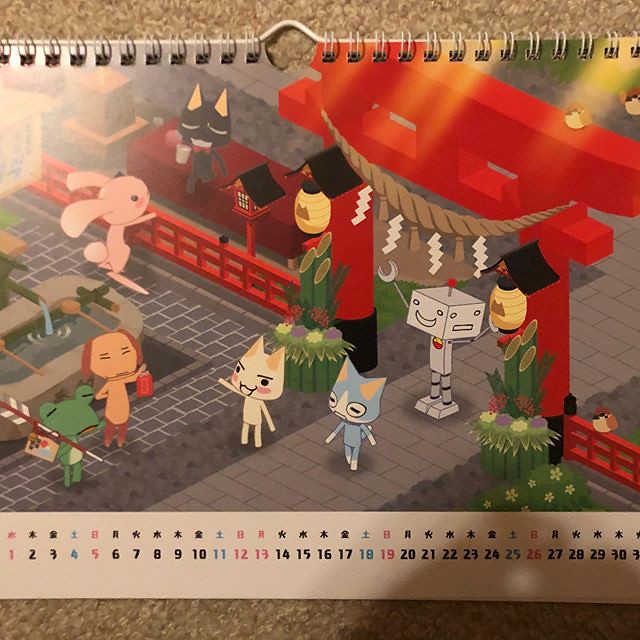This image depicts a spiral-bound calendar page laid on tan carpet, displaying a vibrant and detailed illustration primarily inspired by Japanese cartoons. The focal point of the illustration features a red torii gate adorned with paper lanterns, set within a brick courtyard. Surrounding the gate are an assortment of whimsical characters, including cat people, a green frog, a balding man holding a lamp, a rabbit, and a distinctive robot with a rotating head showing different expressions. Along the bottom of the page, the days of the month, numbered 1 through 31, are aligned sequentially, each accompanied by Japanese symbols in primary colors—some numbers in red, some in black, and some in blue—likely indicating weekends, workdays, or holidays.